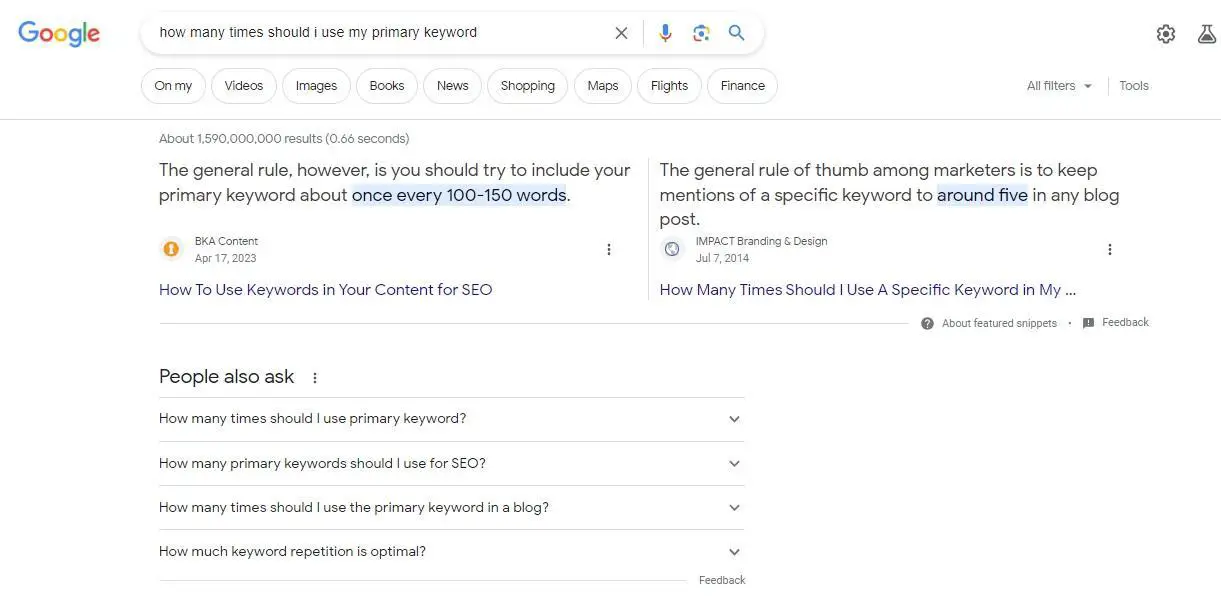The image displays a Google search results page where the user inquired about the optimal frequency for using their primary keyword. The highlighted text response states, "The general rule is you should try to include your primary keyword about once every 100 to 150 words." Adjacent to this, another response mentions, "The general rule of thumb among marketers is to keep mentions of a specific keyword to around five in any blog post." Below the first response, there's a suggestion: "How to use keywords in your content for SEO." Another incomplete suggestion reads, "How many times should I use a specific keyword in my..." without finishing the sentence. Other related questions offered by Google include: "How many times should I use a primary keyword?", "How many primary keywords should I use?", "How many times should I use the primary keyword in a blog?", and "How much keyword repetition is optimal?"